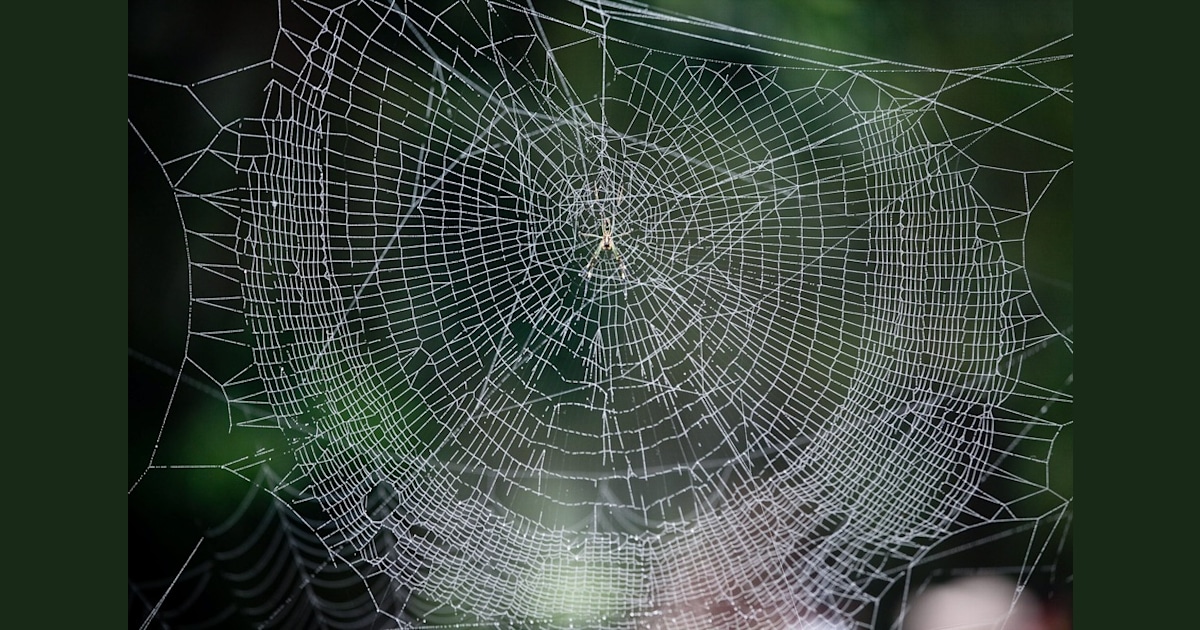The full-color, horizontally rectangular photograph captures an outdoor daytime scene. The image is actually square and positioned within a green border on both the left and the right sides. The background features blurred green vegetation, providing a natural, softly lit backdrop. Central to the picture is an intricate, circular spider web, meticulously woven with a mix of tighter weaving towards the edges and loosely threaded sections in between, giving it a somewhat abstract appearance. Nestled in the middle of the web is a brown spider, diligently at work. The web itself appears pristine without any caught prey. In the lower right-hand corner, the blurry top of a forehead with dark hair peeks into the frame, adding a subtle human element to the composition.